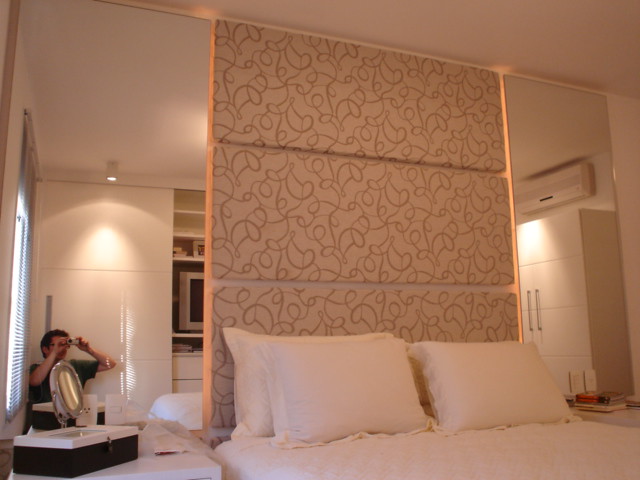This photograph captures a softly-lit hotel room featuring a queen-size bed centrally placed with an ornate headboard that extends from the bed frame to the ceiling. The headboard is richly designed with three large, backlit rectangular cushions adorned with copper swirly patterns, giving it an elegant feel. The room is decorated in a cohesive white color scheme, including large white pillows and sheets. To the side, a white armoire and an end table with a mirror are present. Mirrors are mounted on the sides of the headboard, reflecting a man sitting cross-legged in the corner by a window with sunlight streaming through. The overall ambiance of the room is serene and sophisticated, enhanced by the intricate details of the headboard and the soft lighting.